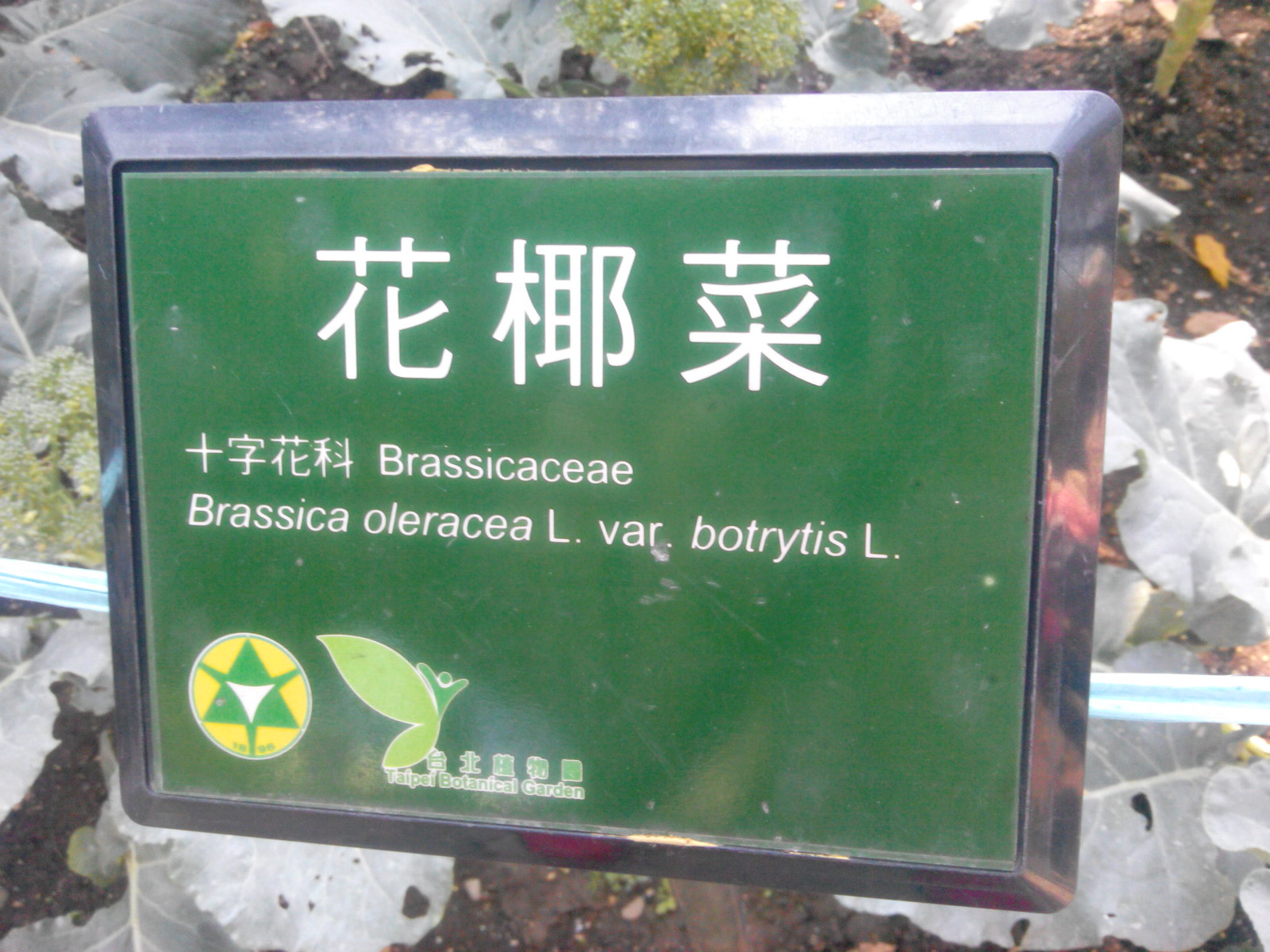In a verdant outdoor setting featuring lush greenery and various types of leaves, there is an informational sign mounted amidst the plants, suggesting a park or garden exhibit, likely at the Taipei Botanical Garden. The sign is framed with a reflective silver border and features a dark green background. At the top of the sign, white text in Japanese provides information, alongside Latin scientific names such as "Brassica casei" and "Brassica oleracea var. botrytis L." Towards the bottom, there is a sticker that includes a white-outlined circle with a yellow interior, a green triangle with radiating green lines, and a smaller white triangle. Additionally, a green leaf symbol is present. The sign incorporates multiple languages, indicating its educational purpose in a multicultural environment. The backdrop reveals a mix of medium to dark green foliage, including notable ruffly leaves, enhancing the vibrant natural ambiance.